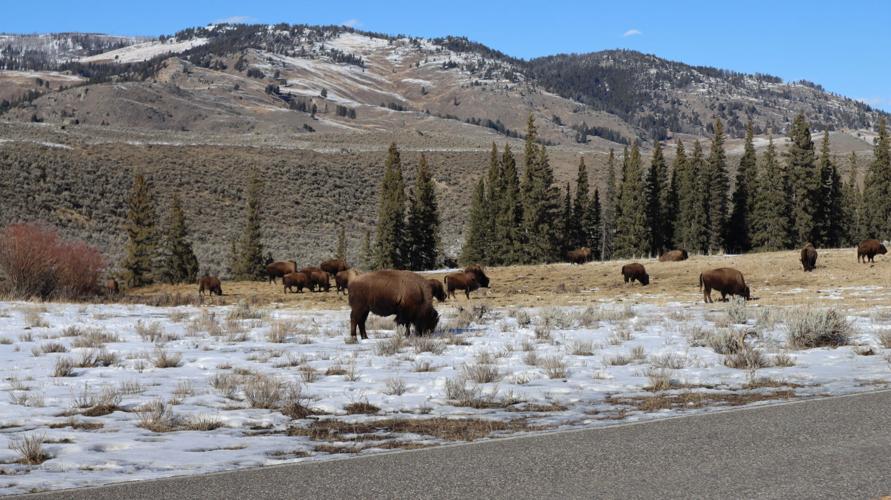The image depicts a serene scene likely taken at Yellowstone during early spring, characterized by a mix of melting snow and emerging brown vegetation. Under a bright, clear blue sky without clouds, sunlight illuminates the landscape. In the background, two mountains, one potentially a low-rise ski hill, have patches of snow on their slopes. Evergreen trees, tall and reminiscent of Christmas trees, cluster more densely on the right side of the scene, while red brush is notable on the left. Scattered throughout the mid-ground are about a dozen buffalo, primarily grazing on spots of exposed vegetation amidst the snow. A road in the foreground intersects the field where the buffalo roam.